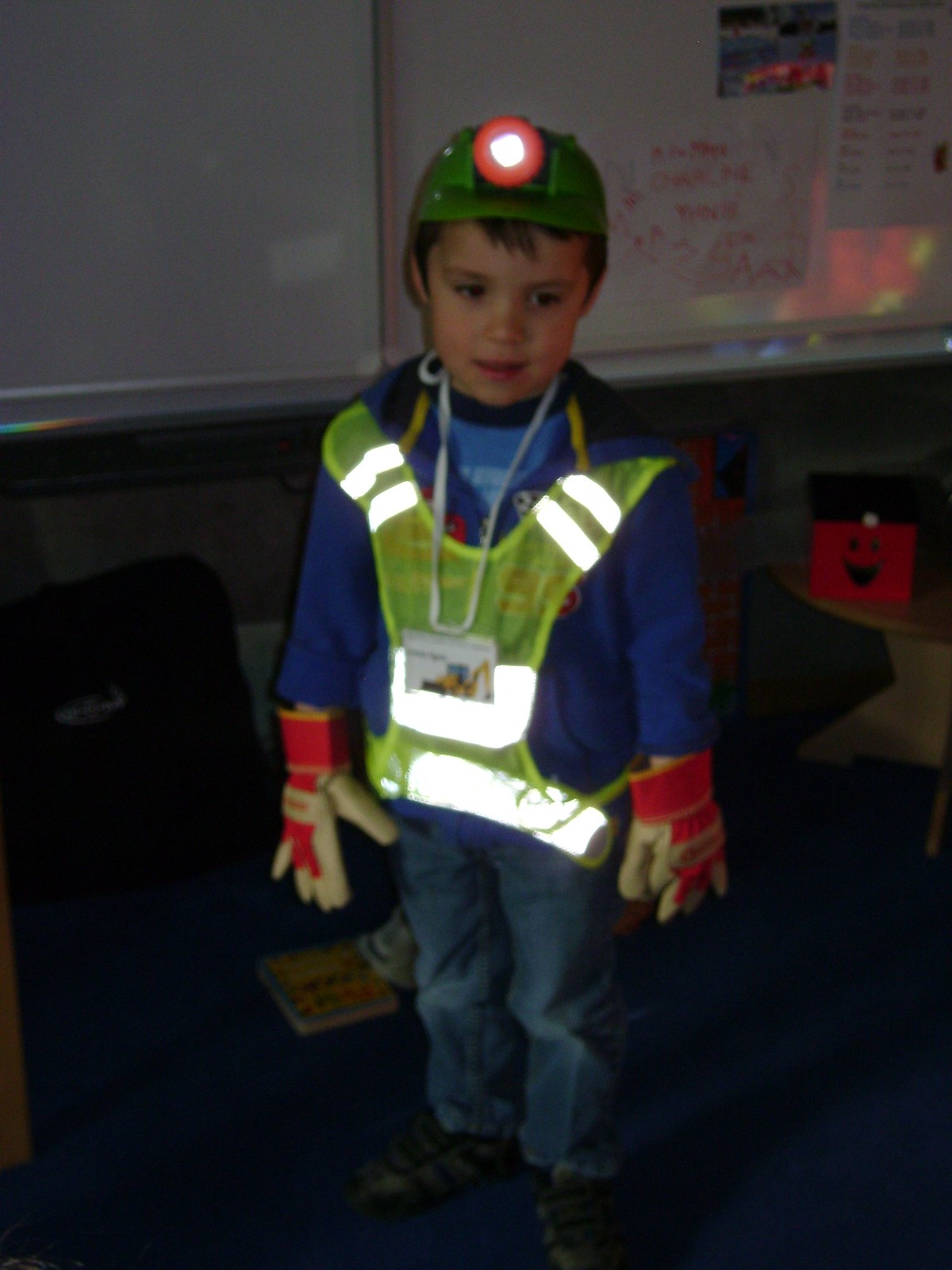A young boy, appearing to be around four to six years old, stands in what seems to be a classroom, possibly indicated by the faintly visible whiteboard behind him. He is dressed in a detailed construction worker costume, complete with a green plastic hard hat featuring a red, lit-up flashlight on the front. His dark brown hair peeks out under the helmet, and his reflective yellow safety vest shines with white stripes. Over his bright blue jacket and blue t-shirt with a black collar, he also wears a lanyard that holds a white card around his neck. His small hands are donned in red and white work gloves, complementing his blue jeans and brown shoes. Despite his snazzy outfit ready for any play construction job, he doesn’t appear particularly happy, standing with a serious expression on his face. To the right side of the image, about halfway down, a red square with a smiley face can be seen, adding a pop of color to the somewhat dim setting.